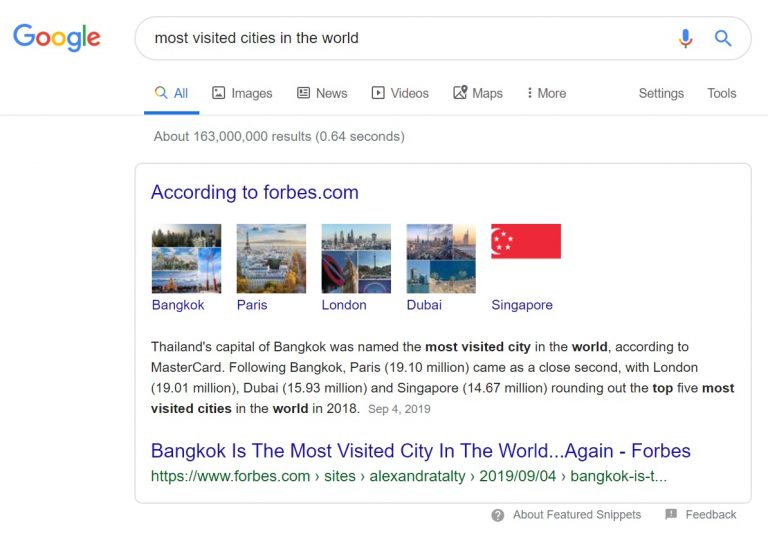A screenshot of a Google search results page is displayed, showcasing Google's multi-colored logo in the top left corner. Beside the logo is the search box with the query "most visited cities in the world." To the right of the search box, there are icons for a microphone and a magnifying glass. Below the search bar are various filter options: All, Images, News, Videos, Maps, More, Settings, and Tools. The "All" option is currently selected, indicated by a blue underline.

Directly beneath the filter options, the page indicates that there are approximately 163 million search results, retrieved in 0.64 seconds. The top result features a snippet from Forbes.com, mentioning five top travel destinations. The cities listed are Bangkok, Paris, London, Dubai, and Singapore. Accompanying images show landmark pictures for Bangkok, Paris, London, and Dubai, while Singapore is represented by its national flag.

Following the snippet, there is a brief description of Bangkok, Thailand's capital city. The first clickable link under this summary reads, "Bangkok is the most visited city in the world again," and references Forbes as the source. The clickable link to the Forbes article appears in green text below the blue hyperlink title.